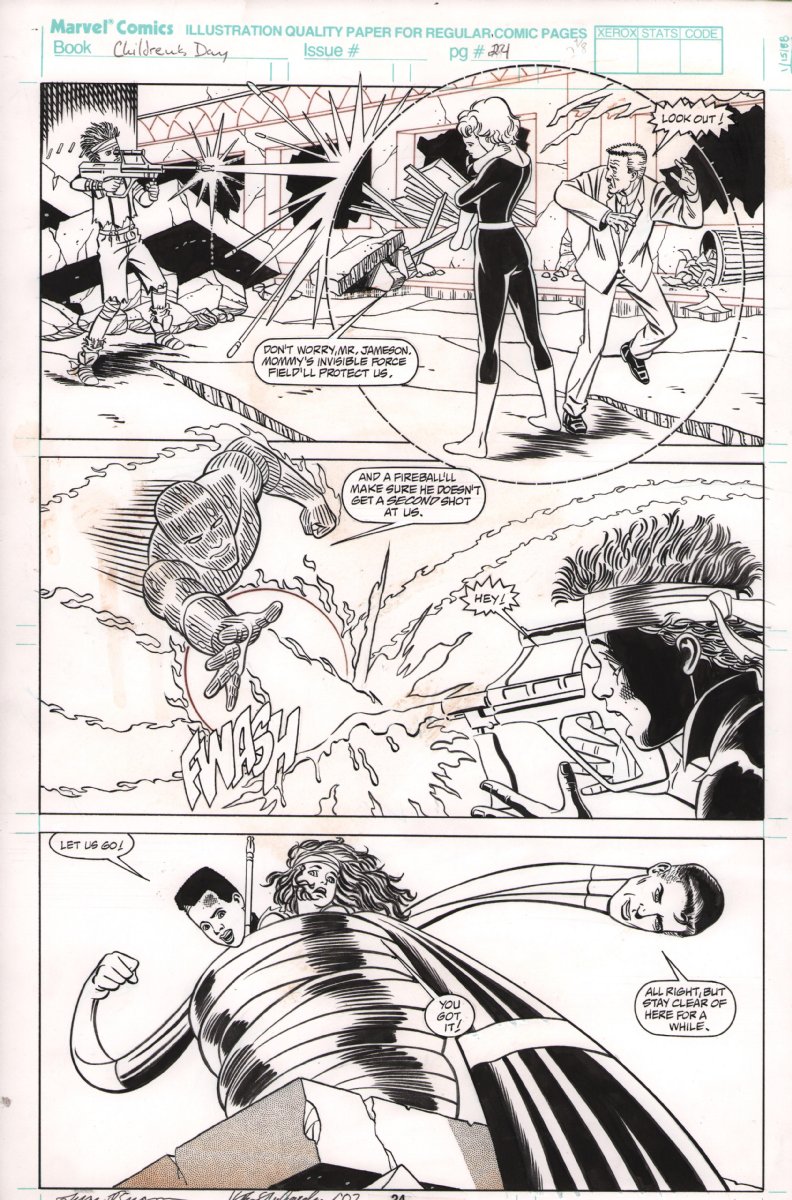This detailed image is a black-and-white comic strip from an official Marvel comic book, specifically page 24 of the Children's Day Issue, which is potentially part of the Fantastic Four series. The top of the page features a banner that reads, "Marvel Comics, Illustration Quality Paper for Regular Comic Pages," with additional notes indicating the book title and page number. 

The comic strip is vertically arranged into three segments. In the first segment, a girl is seen firing a gun at a man and a woman. The woman, likely a superhero, generates an invisible force field around herself and the man to block the gunfire. A dialogue bubble from the woman reads, "Don't worry, Mr. Jameson, Mommy's invisible force field will protect us."

The second segment illustrates the Human Torch flying and launching a fireball at the gun, disrupting the shooter's aim. The text next to him states, "And a fireball will make sure he doesn't get a second shot at us," while the sound effect "FWASH" is prominently displayed, and the shooter exclaims, "Hey!"

The final segment portrays Mr. Fantastic using his stretching abilities to wrap his elongated neck around two individuals, providing them protection. The dialogue in this panel includes a character urging, "All right, but stay clear of her for a while."

The comic strip, with its dynamic illustrations and engaging storyline, emphasizes the protective and offensive maneuvers of the superheroes in the context of a children's special issue.